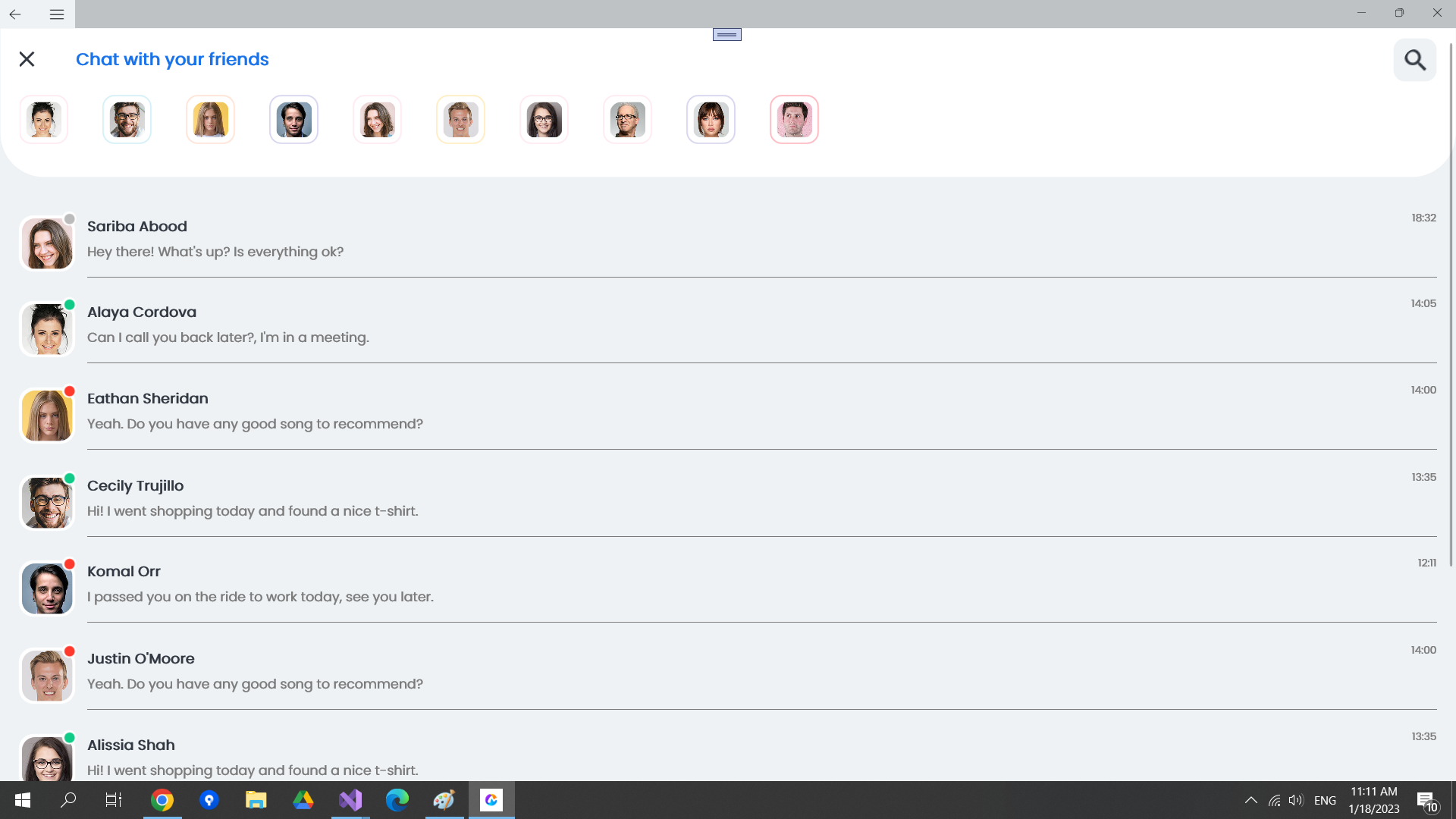A screenshot of a chat application displayed on a Windows operating system (could be Windows 10 or 11) is shown in full screen. The taskbar is visible at the bottom, featuring icons for Chrome, a map application, several folder shortcuts, Google Drive, OneNote, browser options, and the date and time on the far right.

At the top of the chat application, a gray bar contains the title "Chat with Friends," highlighted in blue. Below the title, ten small profile photos of different individuals are aligned horizontally.

The main chat window displays a scrolling list of conversations, each accompanied by profile photos and colored status dots at the top right of the images. Detailed timestamps are visible on the right side of each message. The following conversations are detailed:

1. **Sariba Abood** - "Hey there, what's up, is everything okay?" (grey dot)
2. **Alaya Cordova** - "Can I call you back later, I'm in a meeting." (green dot)
3. **Ethan Sheridan** - "Yeah, do you have any good songs to recommend?" (red dot) - Profile picture of a girl.
4. **Selly Trujillo** - "Hi, I went shopping today and found a nice t-shirt." (green dot) - Appears to be a man with glasses.
5. **Kamal Hoare** - "I passed you on the ride to work today, see you later." (red dot)
6. **Justin Amore** - Repeats "Yeah, do you have any good songs to recommend?" (red dot)
7. **Alicia Shaw** - Repeats "Hi, I went shopping today and found a nice shirt." (grey dot)

At the top right corner, there is a search button represented by a magnifying glass icon, which seems to allow users to search within their chats.